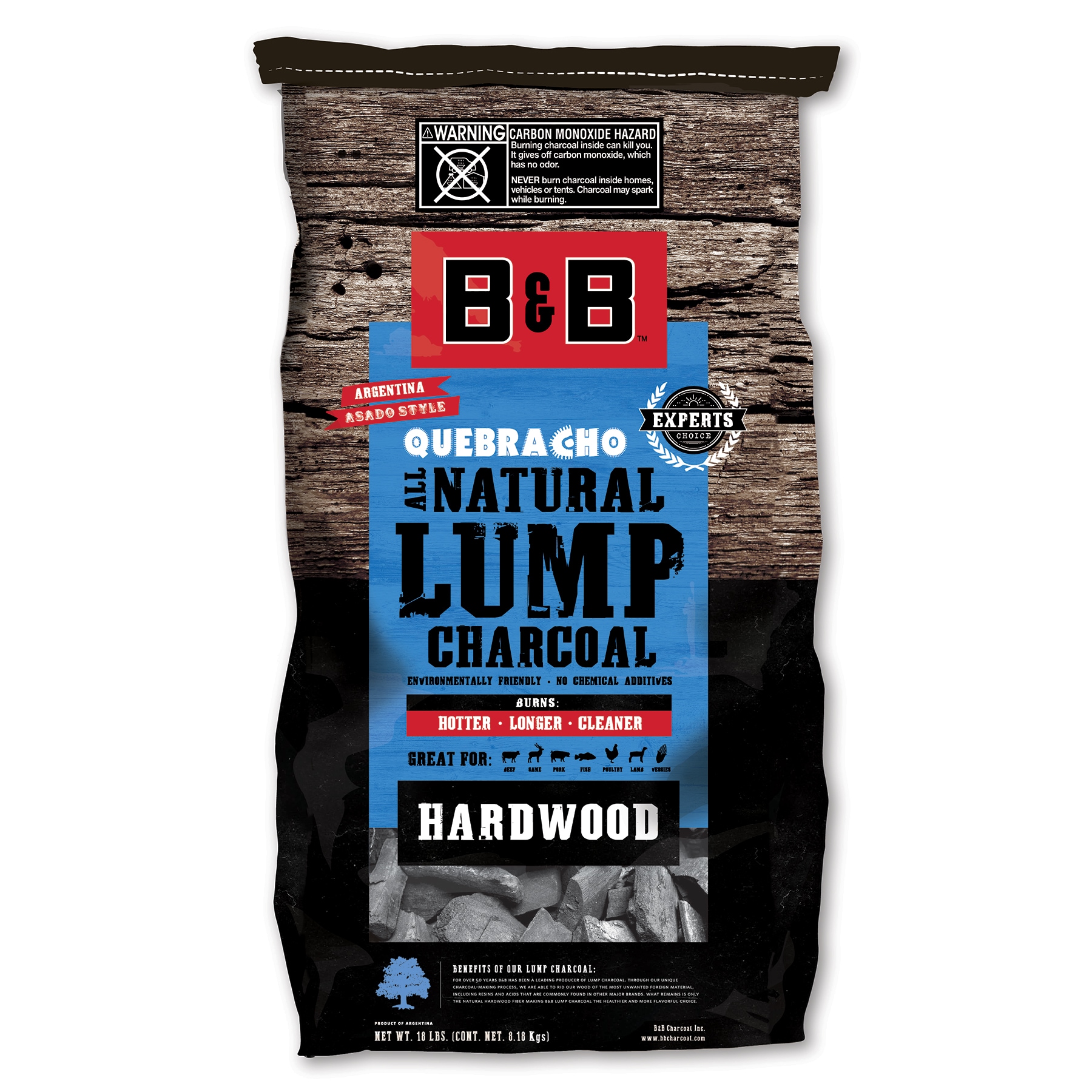The image depicts a bag of B&B Que Bronco All Natural Lump Charcoal designed for barbecue use. The bag features a distinctive two-tone design with a wood-textured brown top and a black bottom. Prominent color accents include red and blue elements. The brand "B&B" is highlighted in red, while "Que Bronco All Natural Lump Charcoal" is displayed prominently. The packaging also specifies that the charcoal is Argentina Asado style. 

A red tag on the front indicates its Argentinian origin, and there is an "Expert's Choice" emblem in black. Notably, the packaging emphasizes that the charcoal burns "hotter, longer, cleaner" and is made from hardwood, which is environmentally friendly and contains no chemical additives. Multiple icons suggest it is suitable for cooking various types of food. A warning label at the top of the bag alerts users to a carbon monoxide hazard. Additional information at the bottom highlights the benefits of using this natural lump charcoal, such as its extended burning time and cleaner smoke profile.